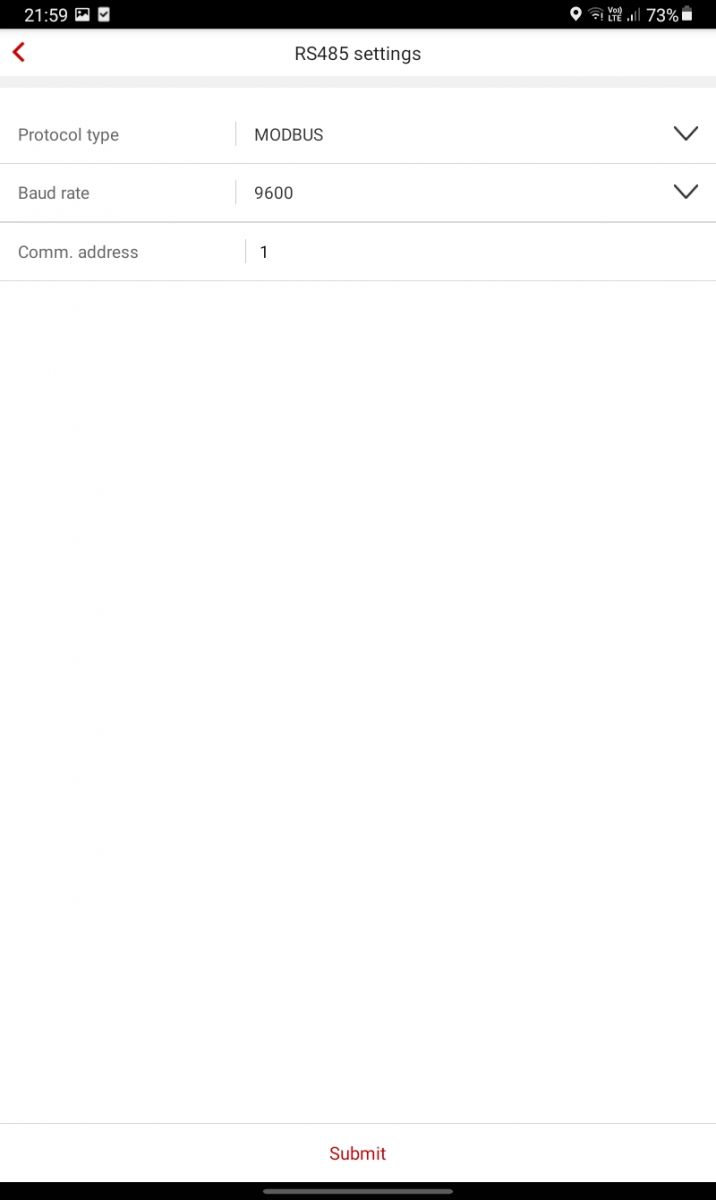The image depicts a minimalist and straightforward smartphone interface. At the top, a black header bar displays the current time, 21:59, along with a battery icon indicating 73% charge, and several typical phone status icons. Below this, a white header section reads "RS-485 Settings" in black text on a white background. A light gray stripe goes across the screen beneath the header, possibly serving as a subtle divider.

Directly below this divider, the interface lists several settings: 
- "Protocol Type," currently set to "MOD-BUS," accompanied by a down arrow for additional options.
- "Baud Rate," set at 9600, also with a down arrow for selecting different rates.
- "COM Address," which is set to 1, but does not feature an arrow for adjustments.

The lower part of the screen is dominated by a large, uninterrupted white space, culminating in the prominently displayed word "Submit" in bold red text at the bottom. This red text stands out against the white background and lacks a surrounding button or distinct clickable area. At the very bottom, a solid black line spans the width of the screen, providing a clear visual endpoint to the interface elements.